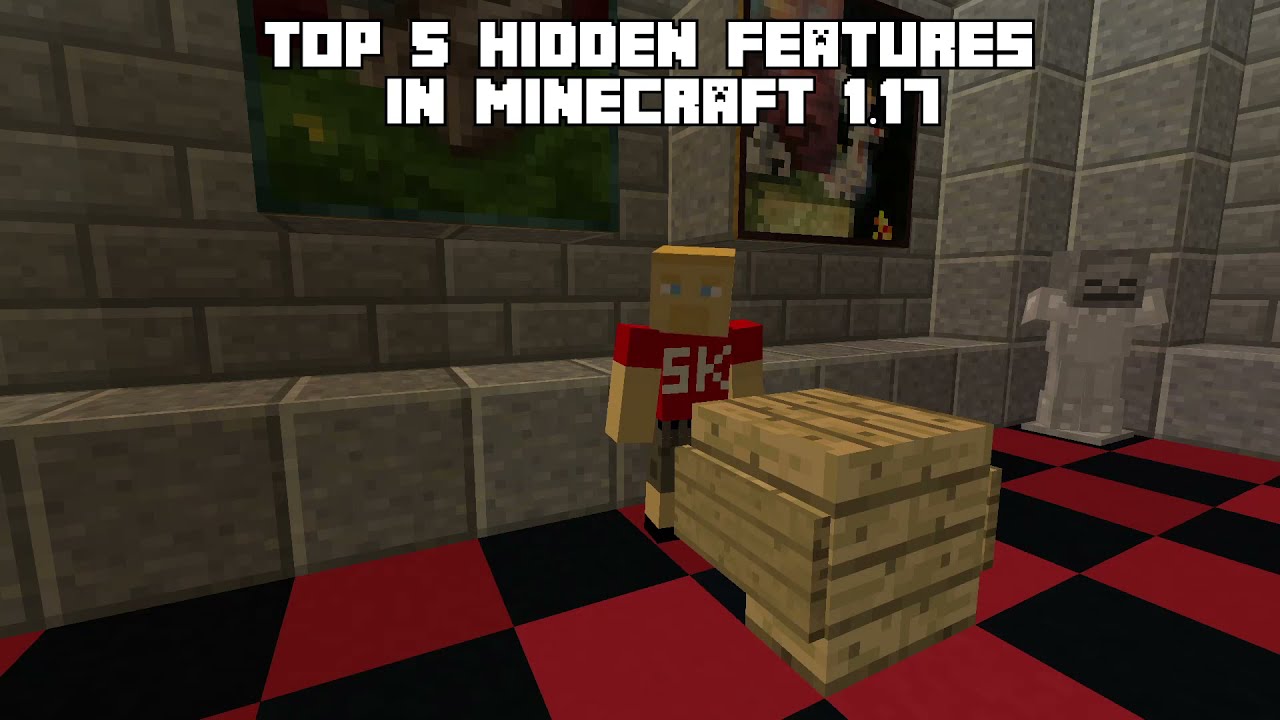The image is a detailed screenshot from an animated video game, likely Roblox, capturing a stone chamber made of large gray and white bricks. The floor of the room is designed with a red and black checkerboard pattern. Centrally positioned on the floor is a large wooden cube. Standing next to this cube is a blocky, Minecraft-like character resembling a Lego figure with a square-shaped head and body. The character wears a red t-shirt emblazoned with "5K" on the front, has tan arms, a square head with blue eyes, black pants, brownish socks, and black shoes. Positioned at the top of the screen in bold white uppercase letters, the text reads "TOP 5 HIDDEN FEATURES IN MINECRAFT 1.17," with each 'A' in the text creatively designed to include a face with eyes and a nose. The character stands in front of stone walls that resemble large cinder blocks, adorned with either framed pictures or window outlines showing scenery in the background. In the corner of the image, a small silvery plain figure with a square head can be seen.